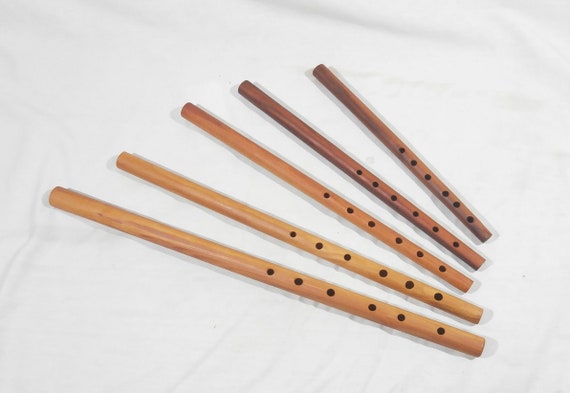The image is a color photograph showcasing five wooden flutes or recorders, neatly arranged on a piece of white fabric with visible wrinkles. Each wooden piece has six holes positioned towards the bottom. The flutes are oriented diagonally, fanning out slowly towards the top left. Starting from the bottom, the longest flute, which is the lightest in color, is positioned closest to the viewer. The pieces vary in color, gradually transitioning from light brown to a deeper burnt orange, and eventually to the darkest brown, which belongs to the smallest flute at the top right. The flutes emit faint shadows on the fabric, adding a subtle depth to the image. There are no people, animals, or structures present in the photograph.